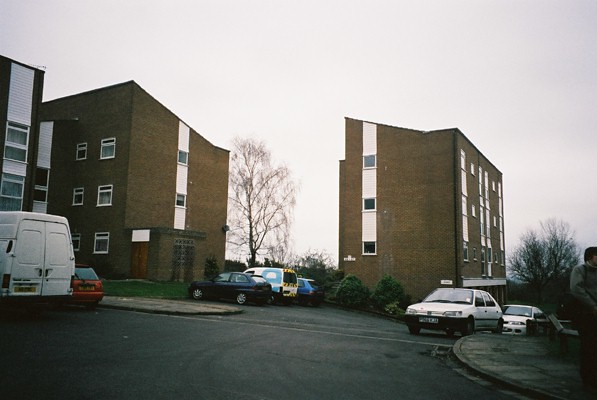This landscape photograph captures a scene of multi-level, brown brick residential buildings with sloped ceilings, situated behind a black asphalt parking lot. Flanked by slightly raised, light gray cement walkways, the parking lot features the backside of a white, box-like utility van on the left, and a smaller red car beside it. Further to the right and scattered across the lot are various other vehicles, including blue and white sedans and an additional white transit van. The gray, overcast sky above suggests a dreary day, contributing to the image's almost nostalgic, possibly timeless feel. The grainy quality of the photo and the vintage appearance of the cars hint that the image may have been taken in the 1990s or earlier. Sparse foliage and trees are visible in the distant background, further framing the scene as a quiet, perhaps almost abandoned, urban snapshot.